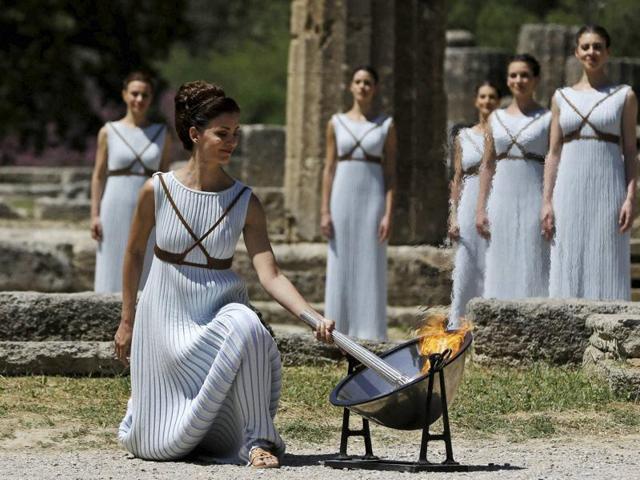In the landscape-oriented image depicting a ceremony, six women dressed in white gowns are present. Their dresses, made of a sweater-like material, feature black holster-like straps crisscrossing over their shoulders and under their ribcages. These women, all seemingly white, stand amidst a backdrop that resembles aged or broken stone ruins, possibly a cemetery with numerous gray stones scattered around. The background also includes some trees, adding to the serene yet solemn atmosphere.

In the foreground, a woman with dark hair, styled up, is kneeling on the green grass with dirt patches. She holds a wooden pole with a slightly grayish tint in her left hand, which she is dipping into a brightly burning fire with yellow, orange, and red flames. This fire is contained within a large silver pot with a black rim, supported by a black metal stand. The woman's attire features the same distinctive crisscross straps, giving a cohesive visual theme to the group. Her focused gaze is directed towards the fire, contributing to the ritualistic and ceremonial feel of the scene.